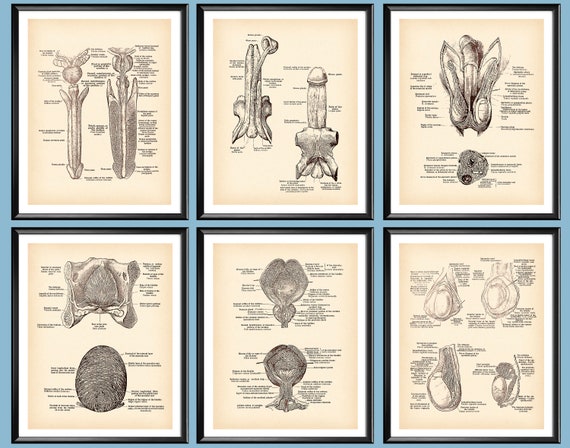The image showcases six detailed scientific illustrations, each framed individually against a blue background. The illustrations are arranged in two rows, with three frames on top and three on the bottom. While all the images are richly labeled, the text is too small to be legible, making it challenging to determine if the subjects are botanical or anatomical. One illustration on the top left resembles the various stages of a seed sprouting, depicting the seed, emerging root, sprouting shoot, and developing leaf structure, eventually showing a root system. The bottom left frame appears to depict something akin to a spinal disc with an ambiguous black oval below it. The illustrations, despite their indecipherable text, collectively exude a scientific aesthetic, suggesting they might be extracts from a science manual, but their exact nature remains elusive.